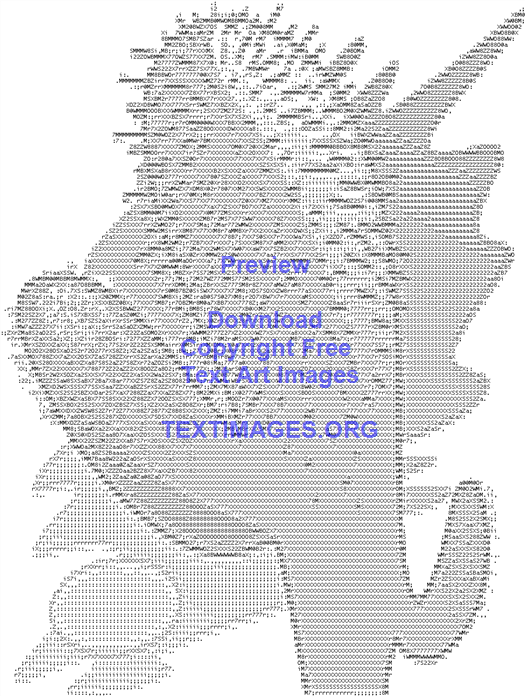The image features an abstract illustration of a cactus, portrayed in shades of gray against a white background. The cactus is detailed with small black lines representing its spines and is composed entirely of tiny text, numbers, and letters, giving it a pixelated appearance. Behind the cactus is a darker gray, textured splotch, adding depth to the composition. Overlaying the image is blue text that reads, "Preview," followed by "Download copyright-free text art images" and "textimages.org." The blue text is centered over the image, which is bordered by a white background.